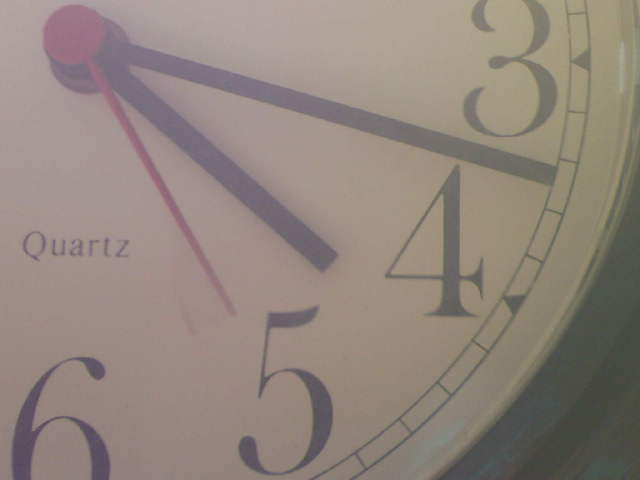This close-up, slightly hazy, black-and-white photo captures the right section of a wall-mounted clock. The clock features a white face with black numbers and minute markers, displaying only the numerals 3, 4, 5, and 6. The clock has three hands: a black hour hand, a black minute hand, and a small red second hand. Centrally placed text reading "quartz" likely indicates the clock's type or brand. The clock is encircled by a gray rim, though the photo's haze makes the white clock face appear somewhat grayish. This is a rather typical quartz clock, possibly found in an office or classroom setting.